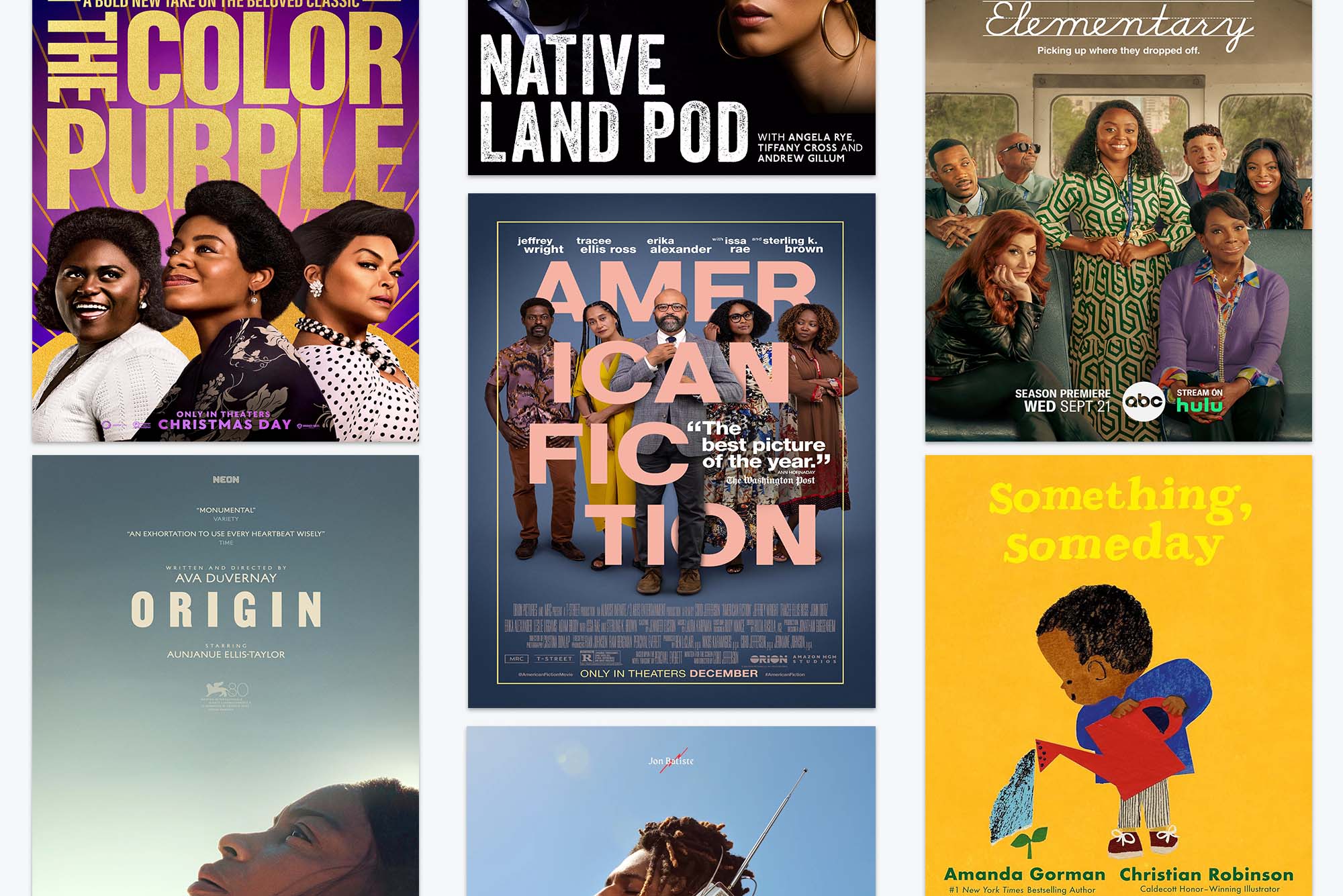The image is a vivid advertisement for a streaming site, showcasing an array of diverse movies and television shows. Anchoring the top left, "The Color Purple" stands out with its purple background and gold text, featuring three proud African American women. Directly below is "Origin," featuring a dark-skinned woman gazing skyward against a gray backdrop. In the middle column, partially cut off, is "Native Land Pod," highlighting the lower part of a woman's face adorned with gold hoop earrings. Below it, "American Fiction" is set against a bluish-gray background and features five individuals, including men in suits and women in dresses. At the bottom, the image cuts off, showing only a blue sky and the top of an African American person's head with a gray antenna-like detail. The right column begins with "Elementary," which shows seven people, the central figure in a green and white dress. Lastly, a vibrant yellow background hosts a cartoon scene from "Something Someday," where a young African American boy with a red watering can and red sneakers waters his dream.